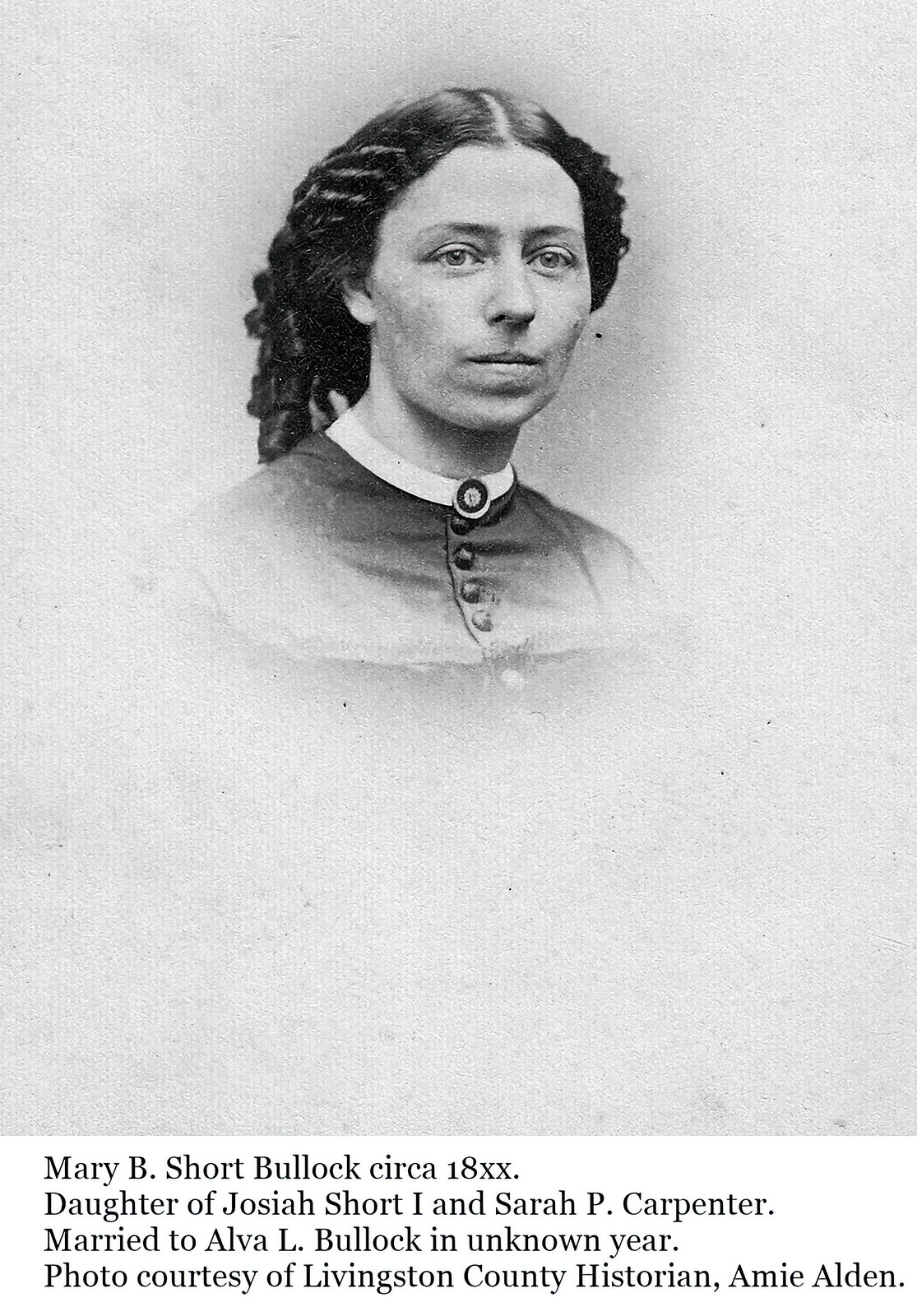This black-and-white photograph, dating from the late 19th century to the turn of the 20th century, features Mary B. Short Bullock, identified as the daughter of Josiah Short I and Sarah P. Carpenter, and the wife of Alva B. Bullock. The portrait captures Mary's face with a serious, stern expression. She appears to have dark hair, which is either braided or curled and falls down her back. Mary is dressed in a high-collared outfit buttoned up to the neck, with a visible white collar and four or five buttons on her dress before the image fades into a white background. Only her head and a portion of her shoulders are clearly visible, as the rest of her body fades out. The photo is credited to Livingston County historian Amy Alden.